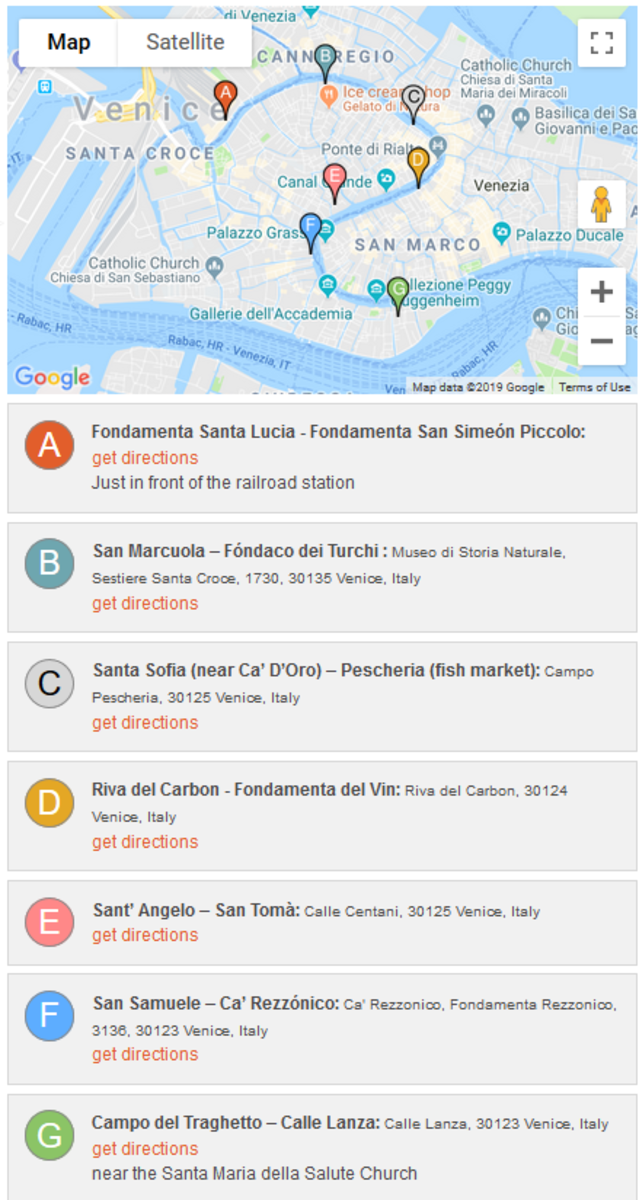This image, captured from a cell phone screen, showcases a detailed map of Venice. The map is displayed in the standard view, highlighting the intricate network of waterways and several marked locations, identified with pins labeled from A to G. 

- **Pin A**: Indicated at the top of the screen as "Fondamenta Santa Lucia / Fondamenta San Simone Piccoli." The label includes a red "Get Directions" link and notes its proximity to the railroad station.
  
- **Pin B**: Located at "San Marcuola / Fondamenta della Tana," with an option to "Get Directions."
  
- **Pin C**: Marked at "Santa Sofia."
  
- **Pin D**: Points to "Riva del Carbon."
  
- **Pin E**: Highlights "Sant'Angelo / Sant'Ambrogio."
  
- **Pin F**: Identified as "Scalzi S. Marcuola."
  
- **Pin G**: Tags "Campo dei Traghetto."

The map interface includes zoom controls (+ and -) to adjust the view. The selectable options for switching to satellite view are also visible, though the current display remains in the map view. This caption provides a comprehensive guide to the specific locations marked on the map of Venice.